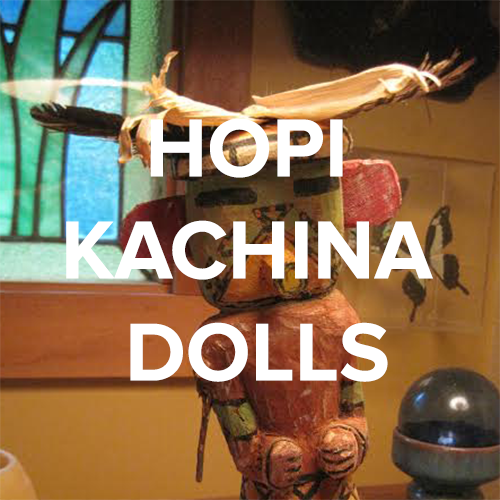The image portrays a detailed museum display featuring a Hopi Kachina doll prominently set against a rich, brown backdrop. The Kachina doll, a traditional Native American wood carving, is adorned with a red hat from which vibrantly hued feathers extend—some brown, some black. Its facial expression, marked by slanted eyes and a lack of a smile, conveys an emotion that might be interpreted as anger or sadness. Green coloring highlights the mid-section of the doll's arms, adding to its intricate design. The statue is encircled by artifacts, including a brown barrel-like vase on the left, and a black and clear globe with a grayish base and a flashing light on the right, enhancing the museum ambiance.

Above the doll, a blue stained glass window decorated with green floral patterns adds a splash of color and illuminates the display. Large white letters in a sans-serif font spell out "Hopi Kachina dolls," capturing the viewer’s attention immediately. Additional background details include various artifacts like butterflies and hints of plants, all contributing to the immersive, cultural atmosphere of the exhibit.